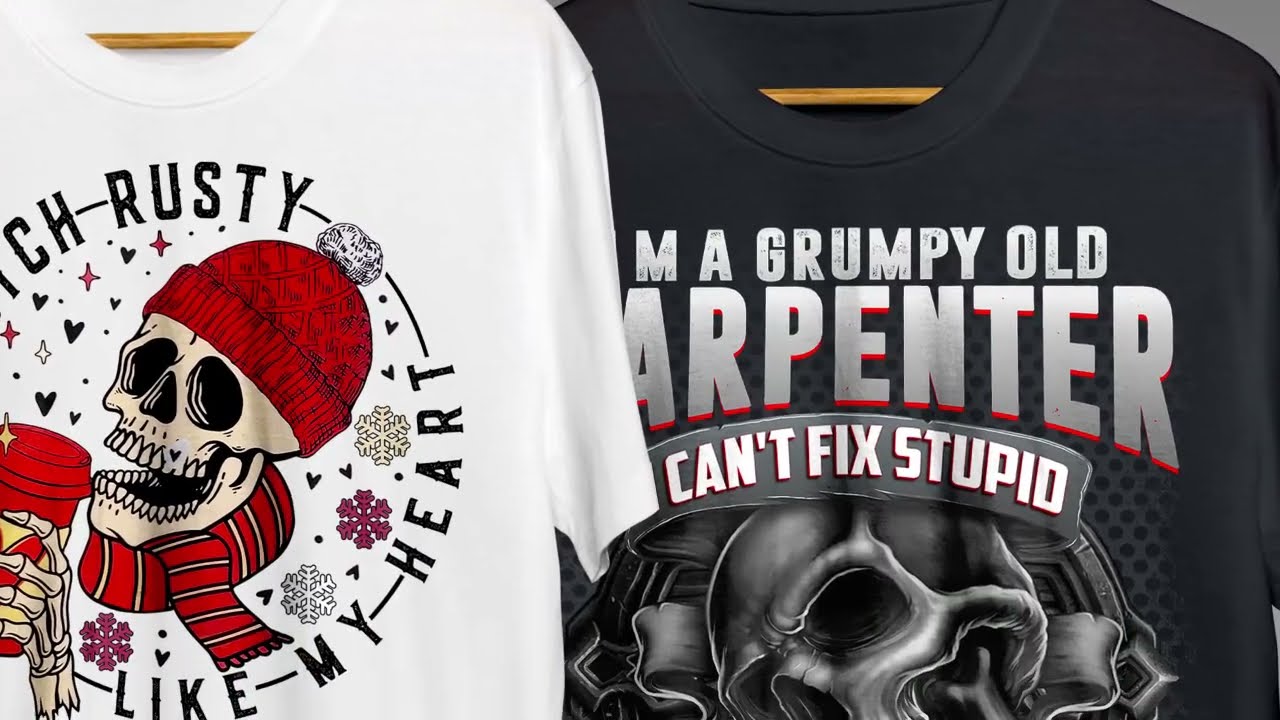This image features two t-shirts hanging side-by-side. On the right, the black t-shirt reads "I'm a grumpy old carpenter who can't fix stupid," accompanied by a partially visible, photorealistic white skull. The shirt is displayed on a brown or yellow hanger. On the left, the white t-shirt showcases a detailed illustration of a skull adorned in winter attire, including a red knit cap with a white pom-pom, a red and white striped scarf, and holding a red cup in its skeletal hand. Surrounding the skull are decorative elements like snowflakes, hearts, and stars. Text encircles the design, partially visible, suggesting a phrase including "rusty" and ending with "like my heart." This shirt also hangs from a similar yellow hanger.